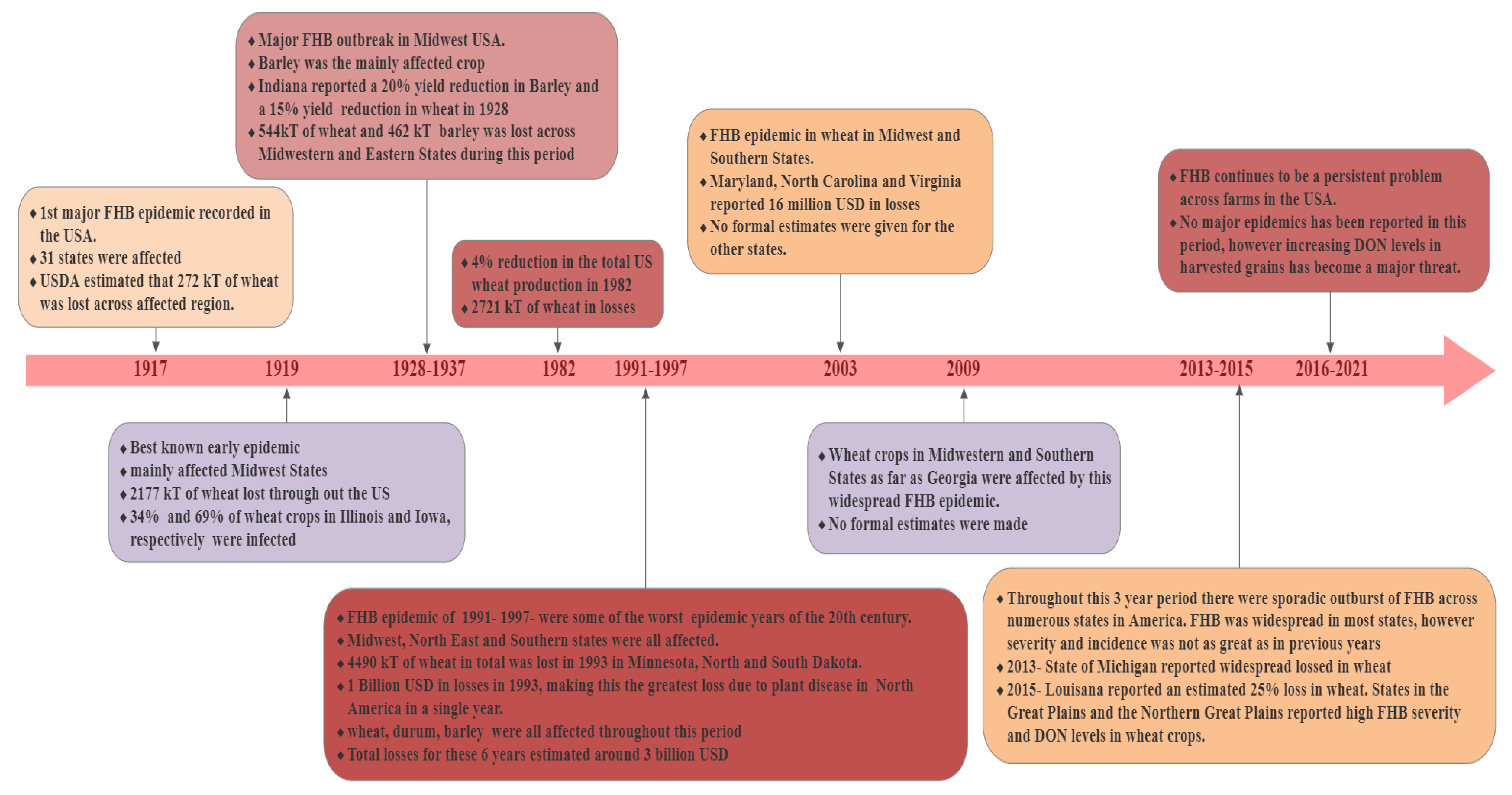The image depicts a detailed timeline spanning from 1917 to the period of 2016-2021, highlighted by a central pink line with an arrow pointing to the right. Surrounding this central timeline are various colored boxes—shades of pink, purple, orange, reddish, and peach—each representing different key events and data points. A significant feature is a large red box at the bottom, detailing the FHB epidemic from 1991 to 1997, which describes it as one of the most severe crop disease events of the 20th century, affecting Midwest, Northeast, and Southern states. The epidemic resulted in the loss of 4490 kilotons of wheat in Minnesota, North Dakota, and South Dakota in 1993, amounting to a financial loss of 1 billion U.S. dollars, marking it as the greatest single-year plant disease loss in North America.

Additionally, the timeline notes the major LFHV outbreak affecting the Midwest USA, with notable impacts on barley and wheat crops. For instance, Indiana saw a 20% reduction in barley yield and a 15% reduction in wheat yield in 1928. Various explanatory boxes with statements and dates hover both above and below the timeline, indicating significant agricultural developments and disease strains that affected crops over the years.